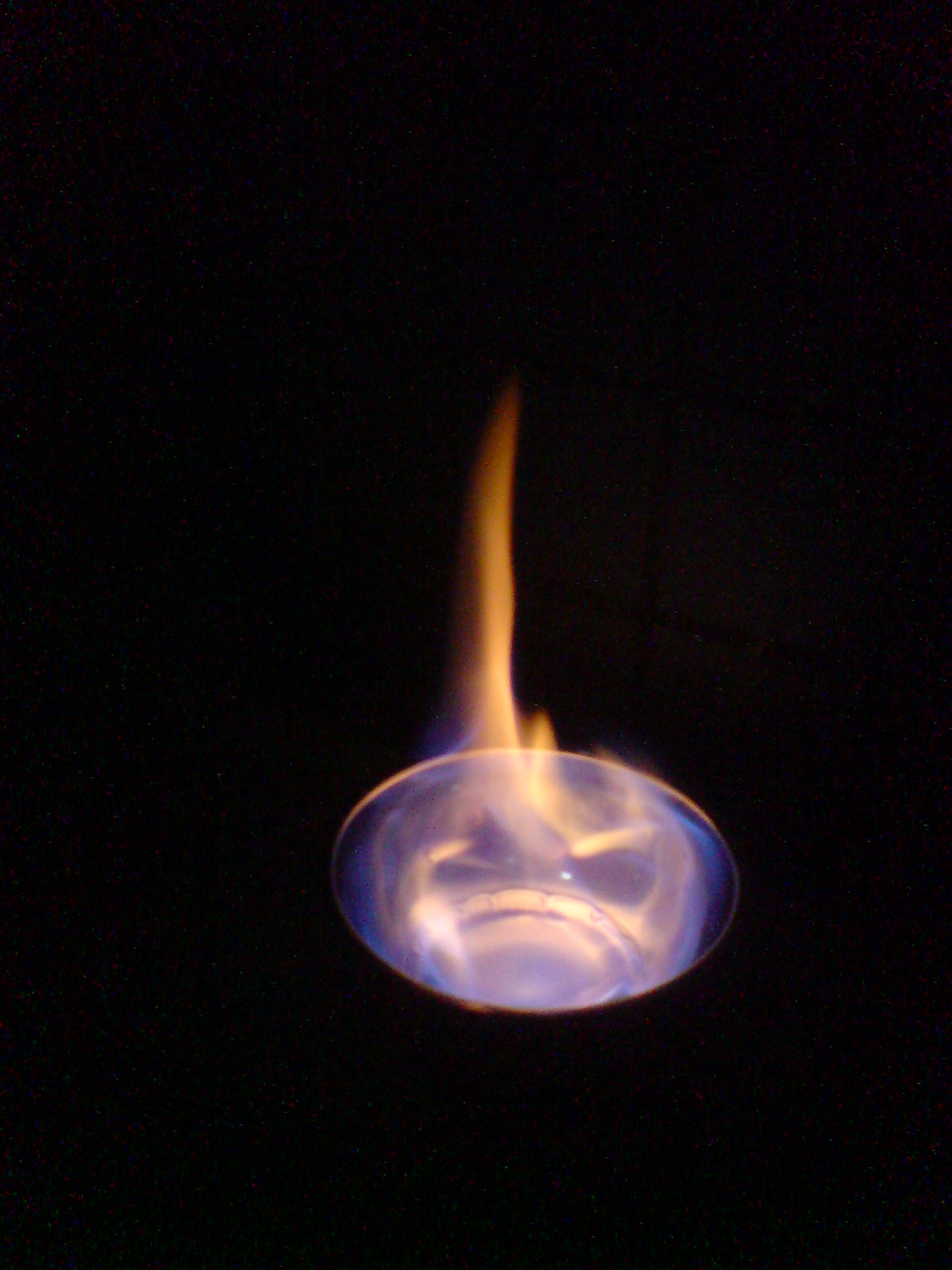The image features a solid black background that extends to all edges of the scene. Positioned slightly above the bottom center is a mysterious oval or circular silver object which appears to have a rim, suggesting it might be a raised dome or a cup. This object is engulfed in fierce flames with distinct color gradations: blue at the base, transitioning to yellow in the higher regions, and orange throughout. The flames create an intense display, with several jagged, smaller flames mingled within the larger blaze. Notably, an intriguing detail within the silver object reveals ambiguous, face-like features, characterized by ominous dark shapes resembling eyes and a downward-turned mouth, enhancing the enigmatic and fiery aura of the scene.